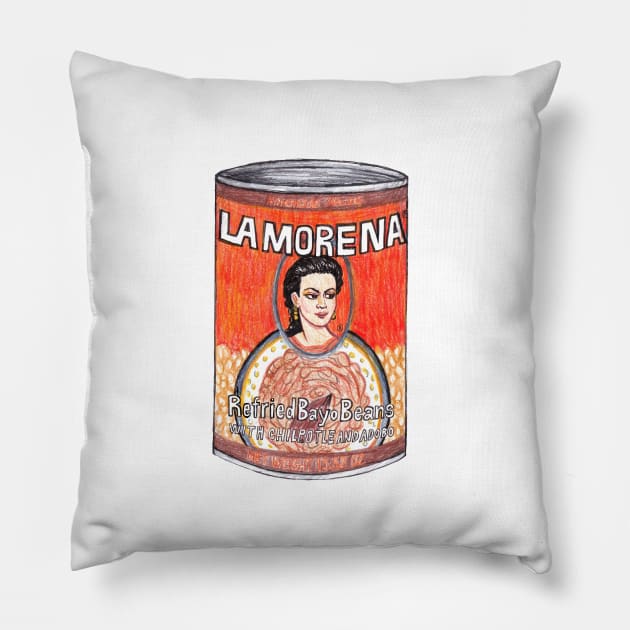The photograph depicts a plain, white throw pillow set against an equally white background. Central to this pillow is a notable hand-drawn illustration of a can, reminiscent of those containing canned vegetables or beans. The can features a predominantly orange top half, capped with a narrow red band. Bold, white capital letters spell out "La Morena" on the orange section, above an oval portrait of a woman with black hair, distinct long earrings, and thin black eyebrows. Beneath her image, the bottom half of the can showcases a bowl filled with what appears to be refried beans, indicated by the text "Refried Bayo Beans with Chipotle and Adobo" inscribed above it. The entire can illustration, strikingly colored with what seems to be colored pencils, adds a quirky, artistic touch to the otherwise plain throw pillow.